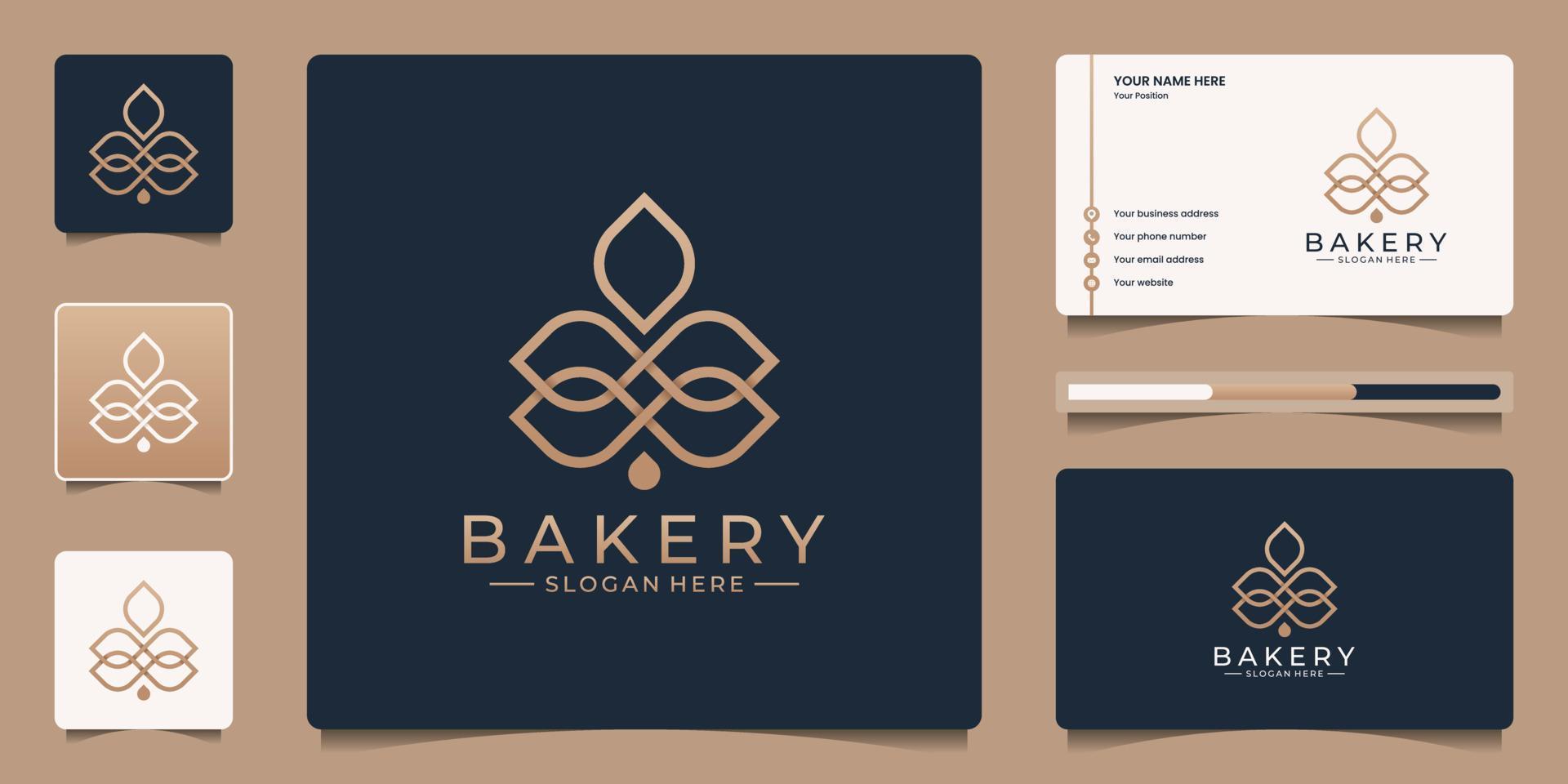This horizontal rectangular image features an advertisement for a company that specializes in creating promotional products for businesses, specifically showcasing various designs for a bakery. The central focus is a brown rectangular card displaying a sophisticated black design with elegant gold text that reads "Bakery" and an editable placeholder for a slogan below it. Surrounding this are smaller versions of the same design in three different colors — white, beige, and black — resembling paper napkins. To the right, there's a business card in white with black and gold elements, paired with a matching card holder. The overall arrangement, set against a tan beige background, highlights the diverse customizable options available for bakery branding, including various sizes and color schemes to suit different preferences.